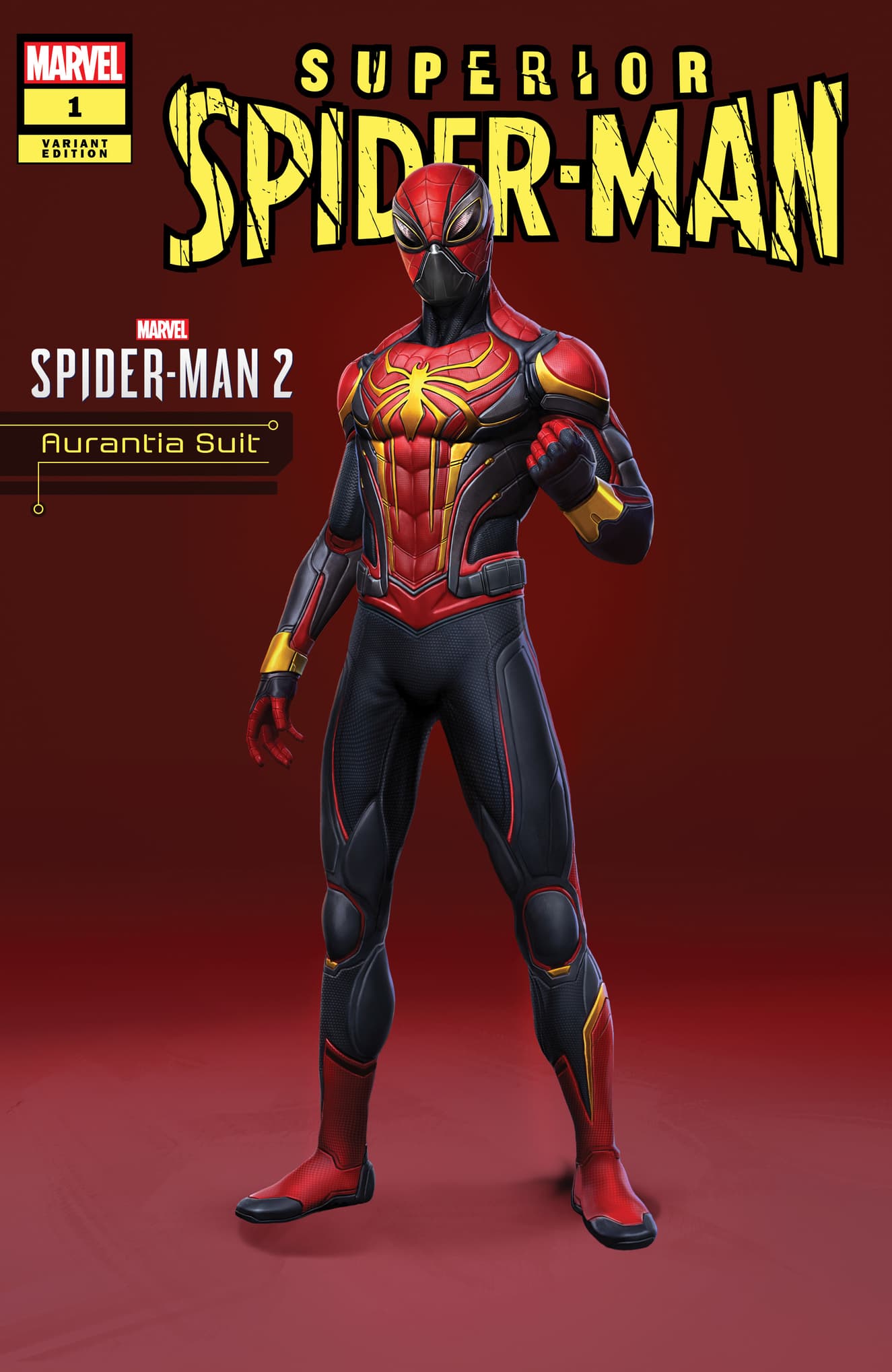This image is a detailed cover of a comic book titled "Superior Spider-Man." At the very top, bold yellow text with a black outline prominently displays the title "Superior Spider-Man." In the upper left corner, the iconic Marvel logo is set against a red background with white text, accompanied by "Number 1" on a yellow background with black text, indicating it's a first edition. Below this, it states "Variant Edition." Another text near the top left reads "Marvel Spider-Man 2: Arantia Suit," highlighting a unique suit variant.

The central figure on the cover is Spider-Man, distinguished by his different attire. His suit is a blend of black and red with notable gold accents, including a golden spider emblem on his chest, golden accent lines down his midsection, and golden bracelets. This Spider-Man’s mask is also black and red with more narrow eye slits compared to the traditional Spider-Man look. His right arm is lowered while his left arm is raised in a fist-pump gesture. The background behind him is a deep reddish hue with shadows, creating a dramatic effect. The overall composition suggests it might be promotional material, possibly for a special edition or downloadable content.